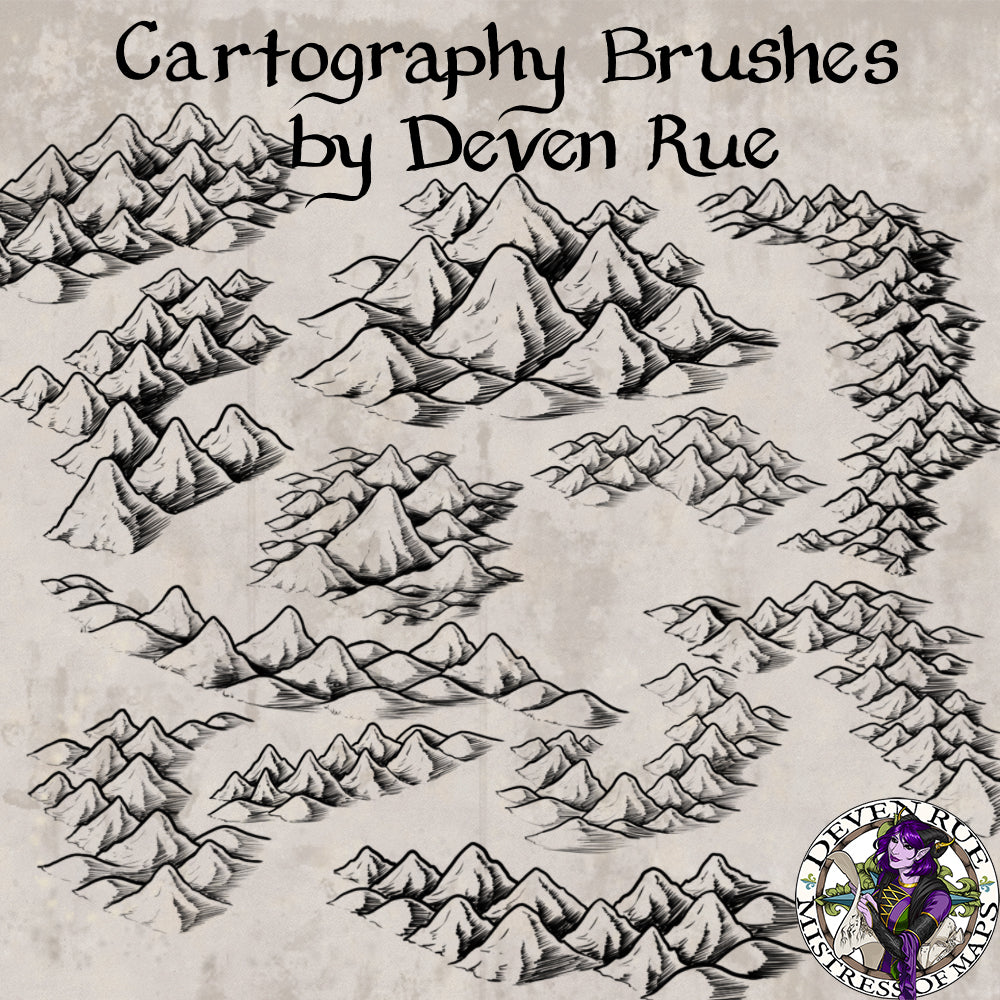The image is a high-quality, black-and-white drawing showcasing a collection of detailed mountain ranges and hills, serving as an example of cartography brushes created by Devin Rue. At the top, it prominently features the text "Cartography Brushes by Devin Rue." The drawing displays a variety of mountain sizes, likely intended to exhibit the range and precision of the brushes, which are designed for digital painting programs like Photoshop, Clip Studio Paint, or Krita. In the bottom right corner, the artist's logo is visible, depicting a woman with pointed elf ears, horns, and purple and black hair, smiling while looking at a map. The logo includes the name Devin Rue, "Mistress of Maps," and a fleur de lis design, affirming the artist's identity and specialty. The meticulous detail in each brush showcases the exceptional quality and uniqueness of these cartography tools.